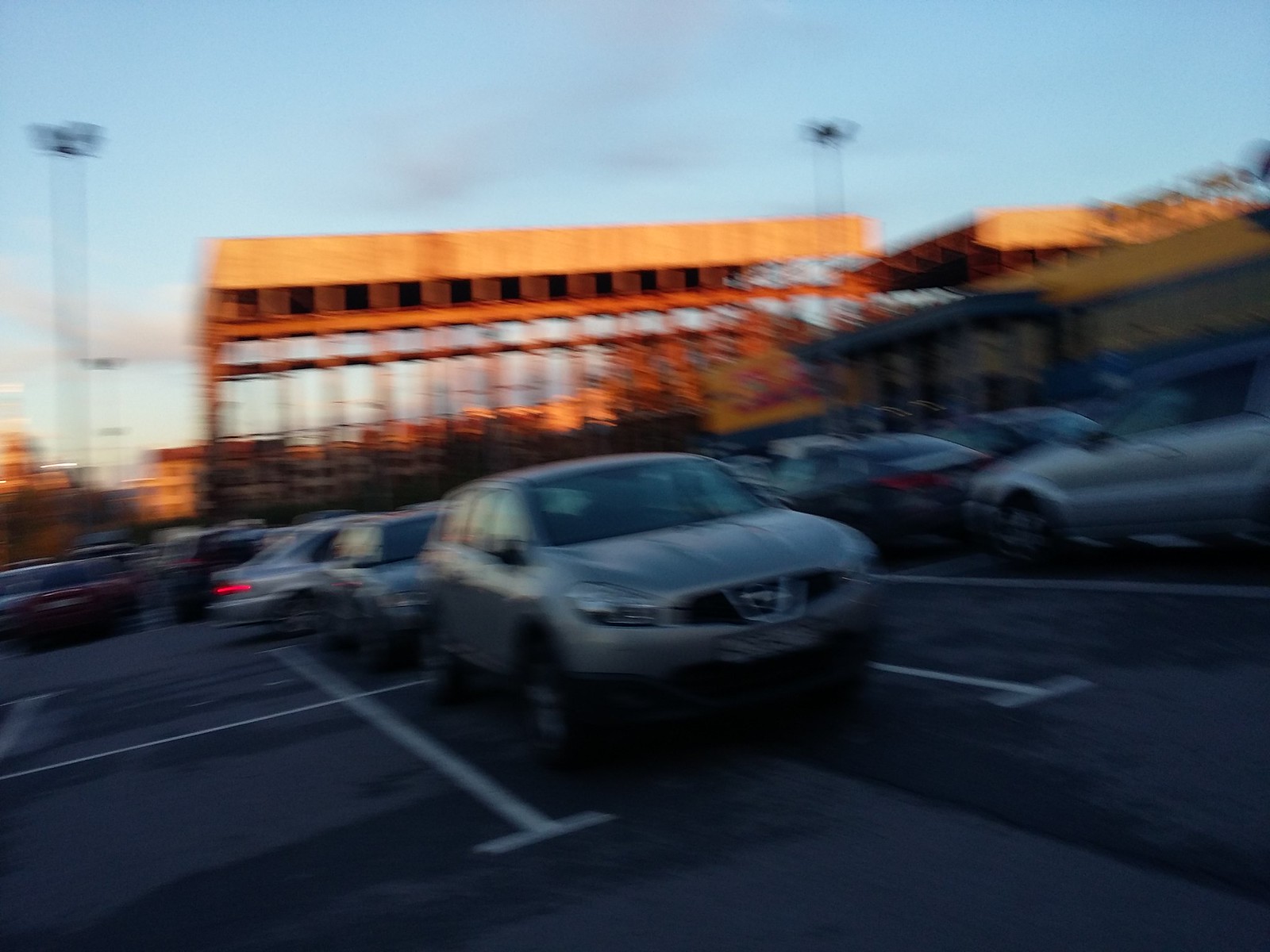The image depicts an extremely blurred exterior scene under natural lighting, focused on a parking lot that appears to be about three-quarters full with cars positioned in various orientations. Dominating the center frame is a silver car with black tires and windows, pointed towards the lower right corner. Parking spots are marked on the ground in white lines. To the right of the image, there's another car, and a third car in the background with its brake light on, indicating it is in motion.

In the background, under a pretty robin's egg blue sky dotted with grayish puffy clouds, there are two tall towers that might belong to an airport terminal. The structure catches the sunlight, exhibiting an orangey glow against the otherwise dimly lit parking lot, which is shadowed, possibly by an unseen building off-frame. Additionally, there's a glassed-in area suggesting an entrance to a nearby building. This building appears to be under construction, with visible wooden frameworks and sections of the roof already completed.